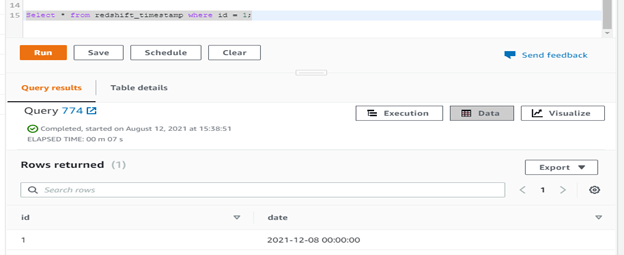This is a detailed screenshot of a computer program interface showing a code editor and query results panel. In the top left corner, numbers "14" and "15" are visible, with "14" written above "15". Adjacent to this, there is SQL code highlighted in blue, which reads: `SELECT * FROM redshift_timestamp WHERE ID = 'L';`. Although the screenshot is partially cut off, a scrollbar indicates more content is available but not visible.

Below this, there is a horizontal row of buttons. The first button, highlighted in orange, is labeled "Run". The following buttons, which are white, read "Save," "Schedule," "Clear," and "Send Feedback" (the latter accompanied by a message icon).

The interface section beneath these buttons is split between "Query Results" (highlighted) and "Table Details". Under "Query Results," it specifies "Query 774," alongside options for "Execution," "Data," and "Visualize," each represented by respective icons – three lines for execution, a dataset for data, and a graph for visualization.

Detailed execution data is provided below these headings. The query was marked as "Completed," with a start date of August 12th, 2021, at 15:38:51. The elapsed time was recorded as 0 minutes and 7 seconds, and one row was returned, as indicated by a checkmark.

Further down, a search bar labeled "Search Rows" is available, followed by export and pagination buttons, and a settings button. The displayed data column headers include "ID" and "Date," showing an ID of "1" and a date of "2021-12-08 00:00:00".